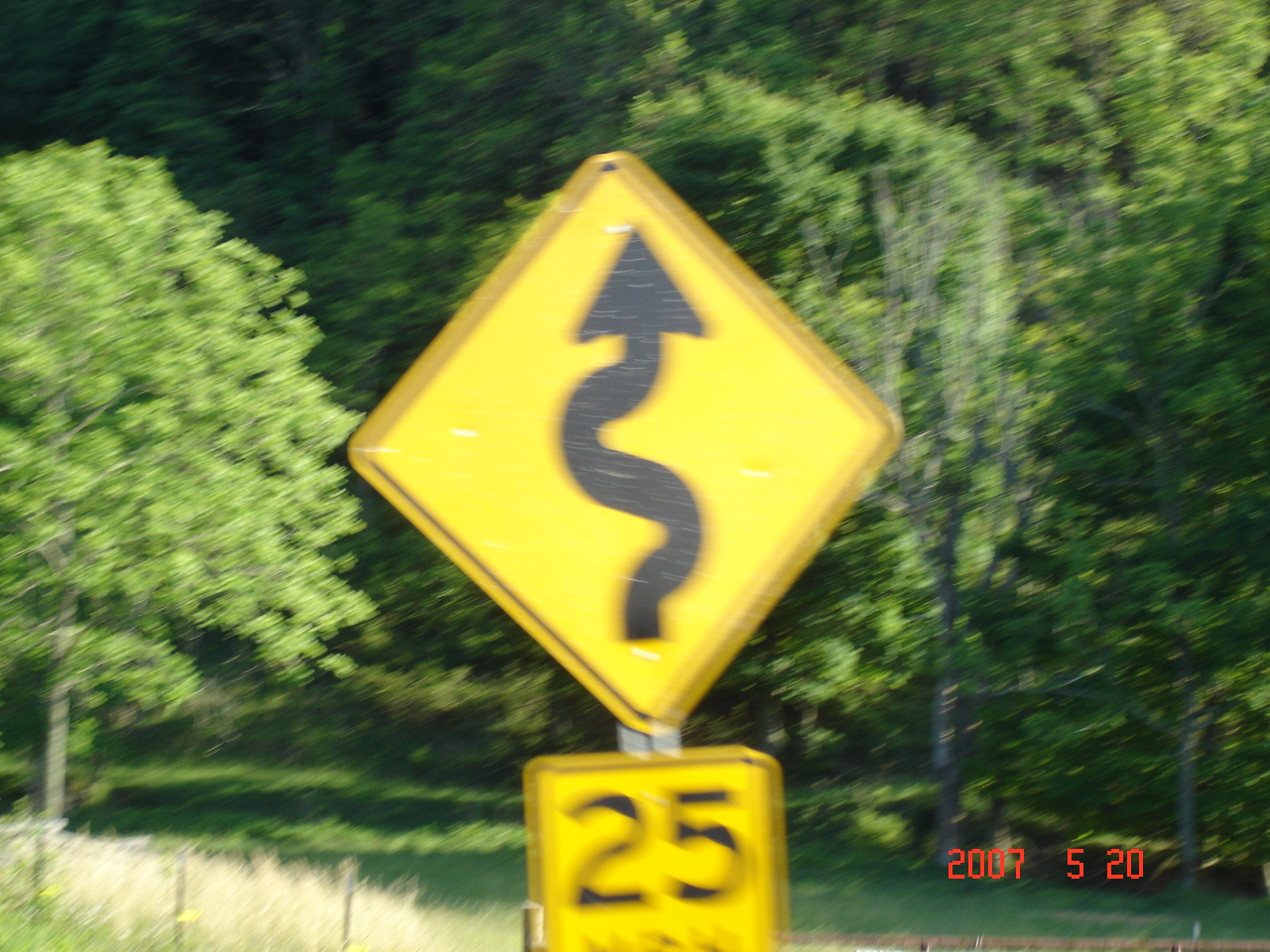In this daytime photograph, a yellow road sign featuring the number "25" is prominently displayed, indicating a speed limit. Above it, a winding road warning sign is visible. In the background, a barbed wire fence stretches horizontally across the image's lower left corner, partially enclosing an area dense with grass and a multitude of trees. The forested area appears dense and extends deep into the woods. The date "May 20th, 2007" is marked in red at the bottom right, adding a timestamp to the scene.